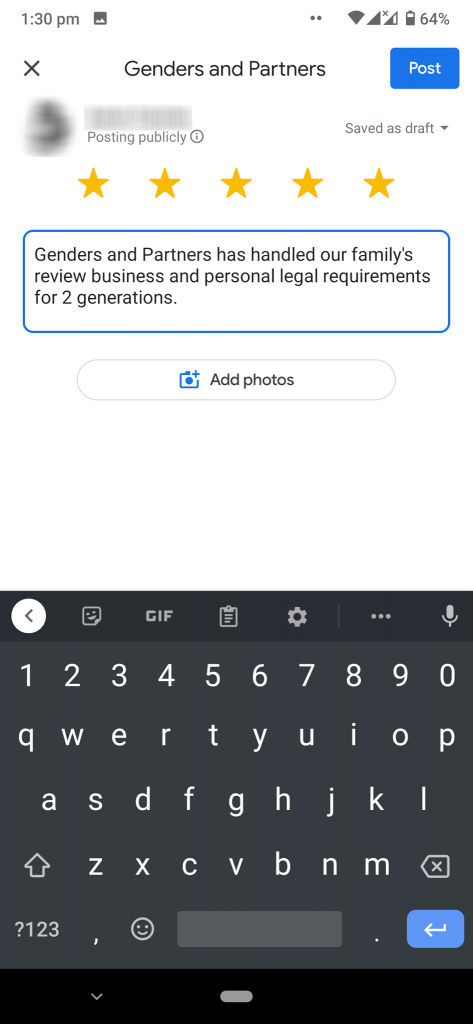This image shows a detailed screenshot of a cell phone rating page for a business named Genders and Partners. The screenshot captures the full cell phone status bar at the top, including the time on the left side, along with the WiFi signal strength, network indicator, and battery meter on the right. Below the status bar, the screen displays the title "Genders and Partners" in black text on a white background, accompanied by a blue "Post" button.

Beneath the title, the page prominently features a five-star rating, followed by a review written by a customer. The review reads: "Genders and Partners has handled our family's review business and personal legal requirements for two generations." Below this text, there is an option to add photos to the review, indicated by a corresponding icon or button.

At the bottom of the screenshot, a virtual keyboard is visible, suggesting that the user is currently in the process of typing or editing their review. The layout of the keyboard is typical of those found on smartphones, used for entering text in various applications. This detailed view encapsulates the entire process of writing and submitting a review on a mobile device.